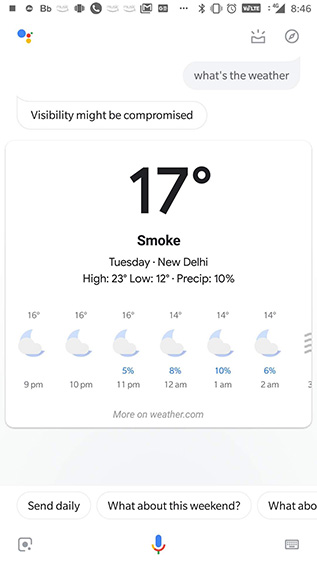In this image, we are looking at a screenshot featuring a variety of icons and text. In the top right corner, the time is displayed as "8:46" in black text. Moving left to right, the text appears slightly blurry, but discernible are a capital 'B' followed by a lowercase 'b'. Adjacent to this text are several icons: a white telephone inside a black circle, the Gmail icon, a cell phone icon, and an alarm clock icon.

In the lower left portion of the screenshot, there's a blue circle enclosing a smaller red and yellow circle. 

In the upper right corner, enclosed in a gray box, black text reads: "What's the weather?" Directly beneath that, in a white box outlined in light gray, black text states: "Visibility might be compromised."

Further down, within a light gray rectangle, a white background hosts large, centered black text displaying "17 degrees." Below this, the text "Bold black smoke" is prominently featured. At the bottom of the image, it reads: "Tuesday, New Delhi, High 23 degrees, Low 12 degrees, Precip 10%."